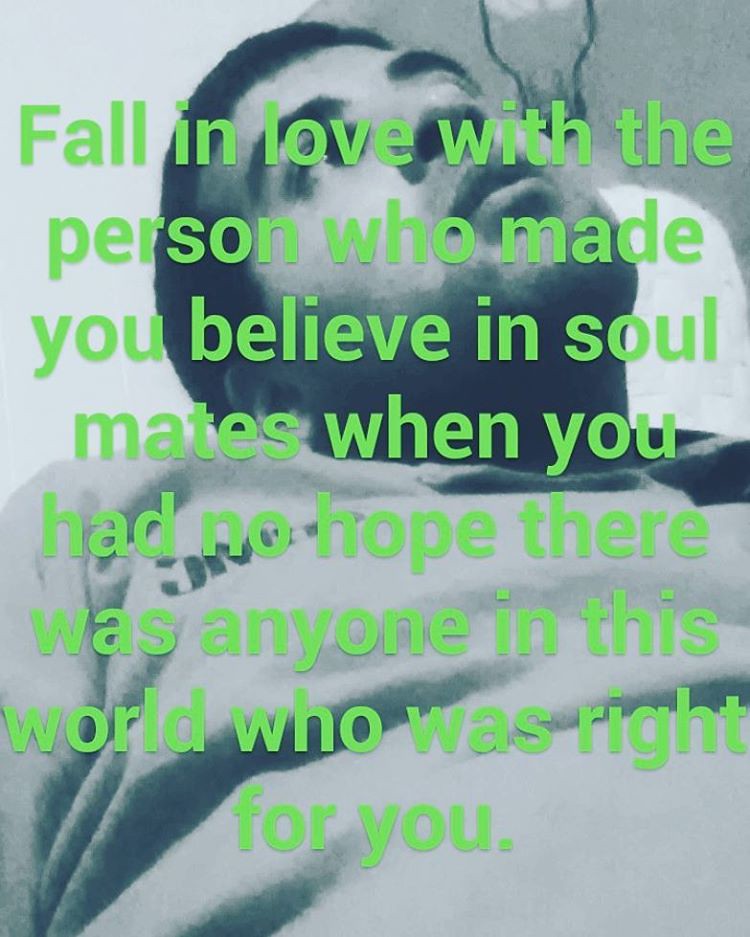The image is a vertically-oriented, black-and-white photograph with a subtle green tint. It features a man with dark hair and a five o'clock shadow, wearing a light-colored sweater adorned with some text that is obscured by both the folds of the fabric and the overlaid quote. The man is positioned in a half-reclining posture, looking upwards to his left with a distant, contemplative expression. His neck is cricked to the right, enhancing his wistful appearance. Dominating the image is an inspirational message in bold, green, sentence-case font: "Fall in love with the person who made you believe in soulmates when you had no hope there was anyone in this world who was right for you." This text covers a significant portion of the photo, adding a reflective and motivational layer. In the background, a blurred object that resembles a lamp adds a touch of domestic context to the setting.